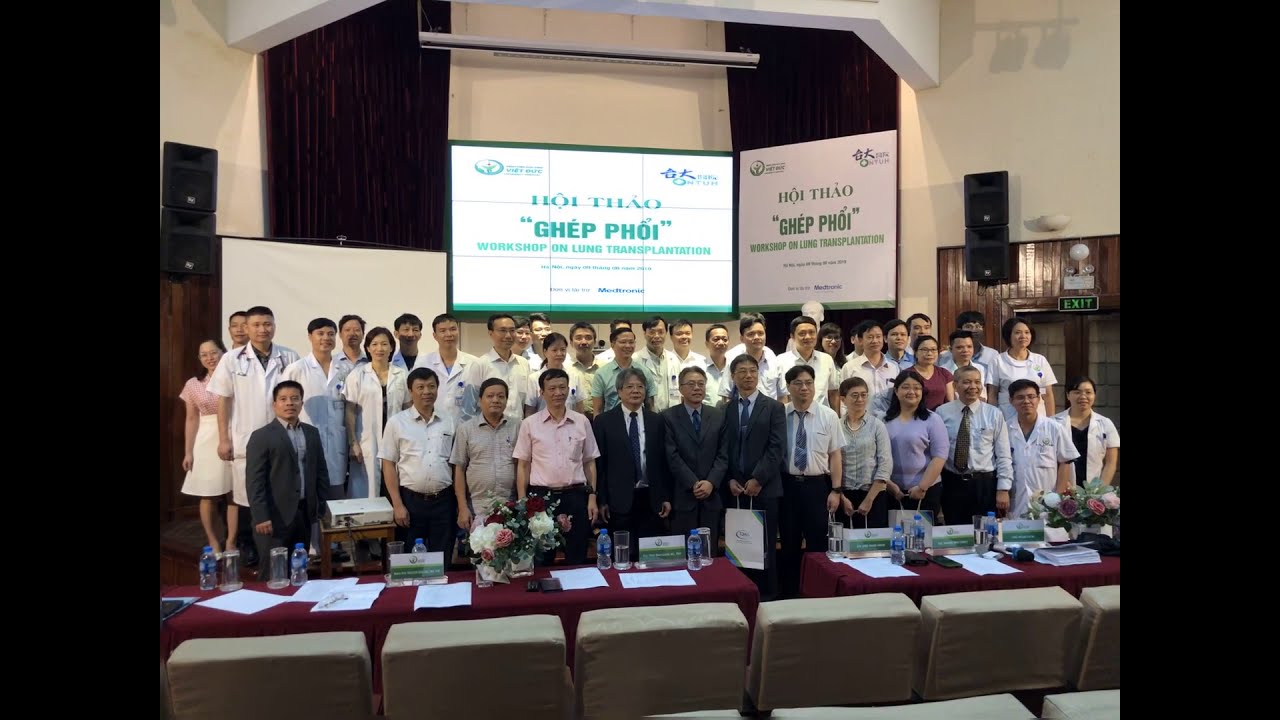The image depicts an indoor conference or workshop, featuring a diverse group of male and female medical professionals posing in front of a podium. The podium is adorned with various monitor or projector signs displaying text in a foreign language, possibly Vietnamese, suggesting the event could be related to lung transplantation or a similar medical topic. In the foreground, there are rows of chairs along with tables lined horizontally, each table set with water bottles, paperwork, and floral arrangements. The attendees are standing together, smiling at the camera, against the backdrop of a large room equipped with speakers and an exit door visible to the right. The setting hints at a formal presentation or award ceremony, with the environment characterized by its indoor ambiance and detailed preparations for the participants. The color palette includes shades of tan, red, white, blue, green, pink, purple, black, and gray, reflecting a vibrant and professional atmosphere.